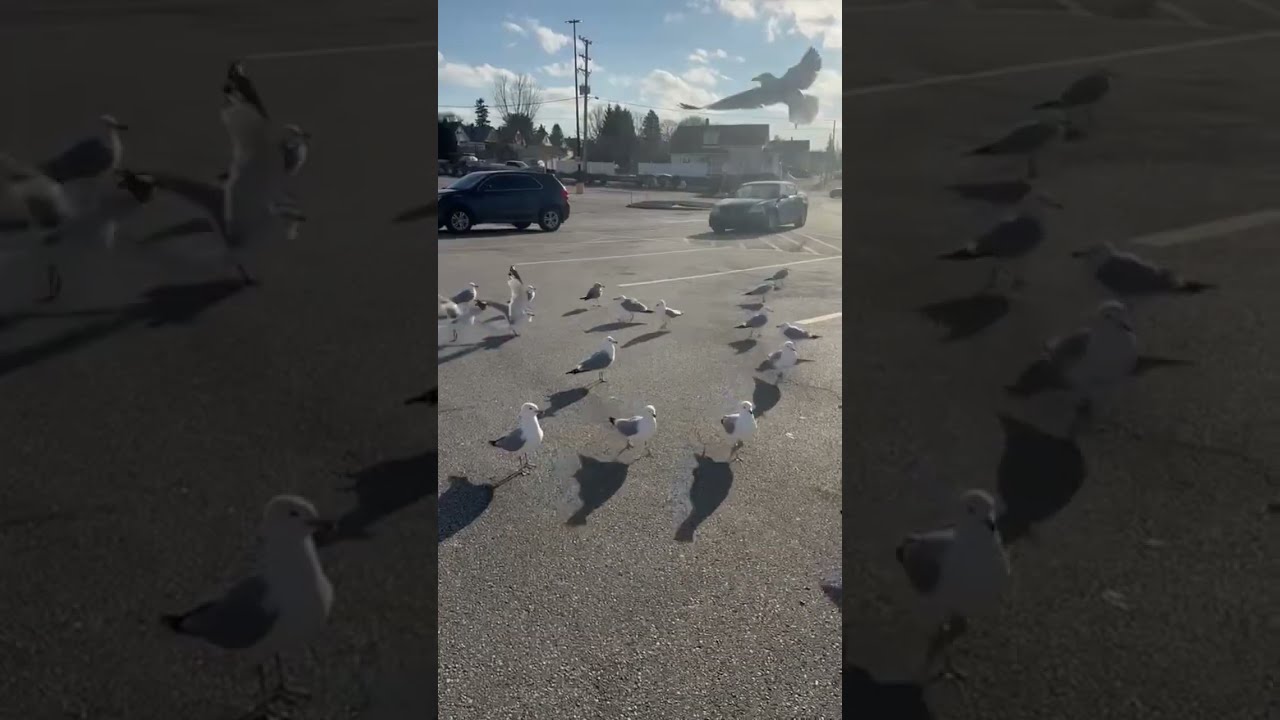The image prominently features a large parking lot bathed in sunlight, with long shadows indicating it might be either early morning or late afternoon. The sky above the parking lot is a light blue with scattered clouds, adding to the sunny atmosphere. 

In the center of the image, a flock of approximately fifteen seagulls, characterized by their white bodies and gray wings, occupy the scene. Most of the seagulls are walking or standing, although one is captured mid-flight, possibly about to land. They are dispersed across the gray asphalt, delineated by white parking lines.

Two vehicles—a gray sedan and a darker-colored SUV—are parked toward the background, not far behind the birds. Further beyond the parking lot, one can see a large white building, evergreen trees, and electrical poles equipped with lights and transformers, with power lines stretching between them.

Interestingly, the photograph has been edited to have a double layer effect, with a vibrant version of the image transposed over a more muted version, emphasizing the flock of seagulls in the middle, centered both horizontally and vertically within the frame. The absence of people in the photo makes the setting appear serene and undisturbed.